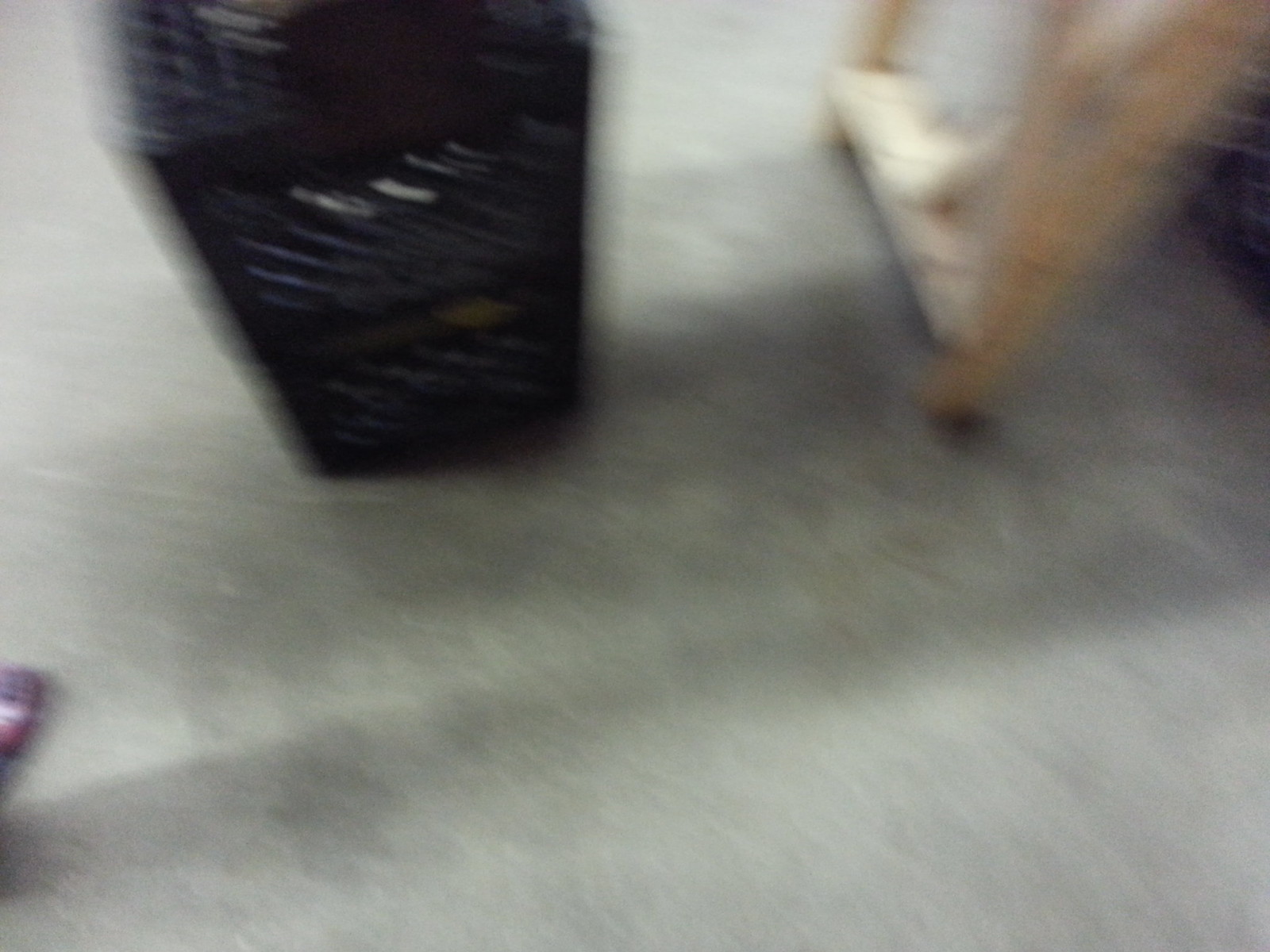This is a blurry close-up photograph taken indoors, possibly in a garage-like space with an illuminated light gray concrete floor. Central in the image are two black, plastic milk crates stacked atop one another. The crates are characterized by holes on all sides and a black object with partially visible white writing is situated on the top crate. To the right, a partial view of a light brown step ladder or desk leg is casting a shadow on the floor. Additionally, there is an indistinct purple object with stripes of pink and red in the lower left corner, possibly illuminated by ambient light, and what seems to be either the shadow of a person or more objects not clearly discernible due to the blur.